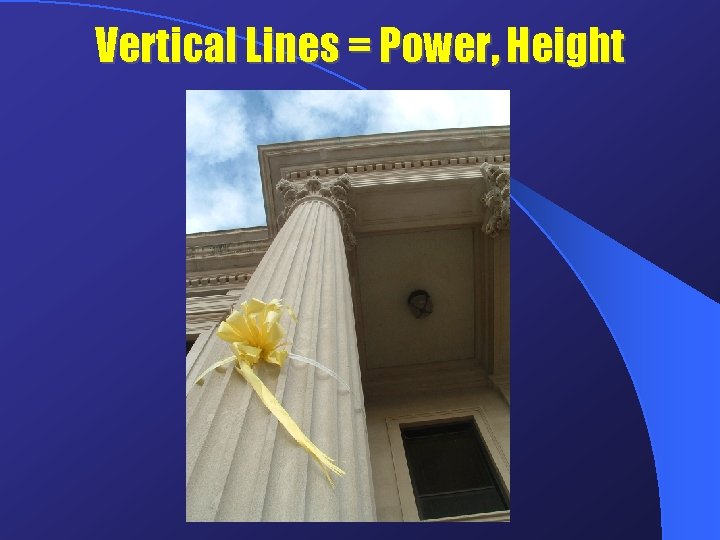The image is a visually striking presentation slide with a central photo and a detailed background graphic. The background features a blue gradient with a wide curved line starting at the bottom right corner and tapering off towards the upper left. At the top of the slide, in bold yellow letters, it states "Vertical Lines = Power, Height."

The central photo captures the architectural grandeur of what appears to be a government building or a structure inspired by Greek architecture. From the perspective underneath the roof, a tall stone column, wrapped with a yellow ribbon and bow, stands prominently to the left. The column exudes strength and sophistication, akin to those found in courthouses or similar edifices of justice and authority. The roof supported by these pillars is clearly visible.

Additionally, there is a black vertical rectangular window located to the right side of the column. Above the roofline, the sky is visible, featuring hues of blue with scattered white clouds, contributing to the serene yet powerful ambiance of the image. The combination of these elements in the slide emphasizes the themes of verticality, power, and architectural elegance.